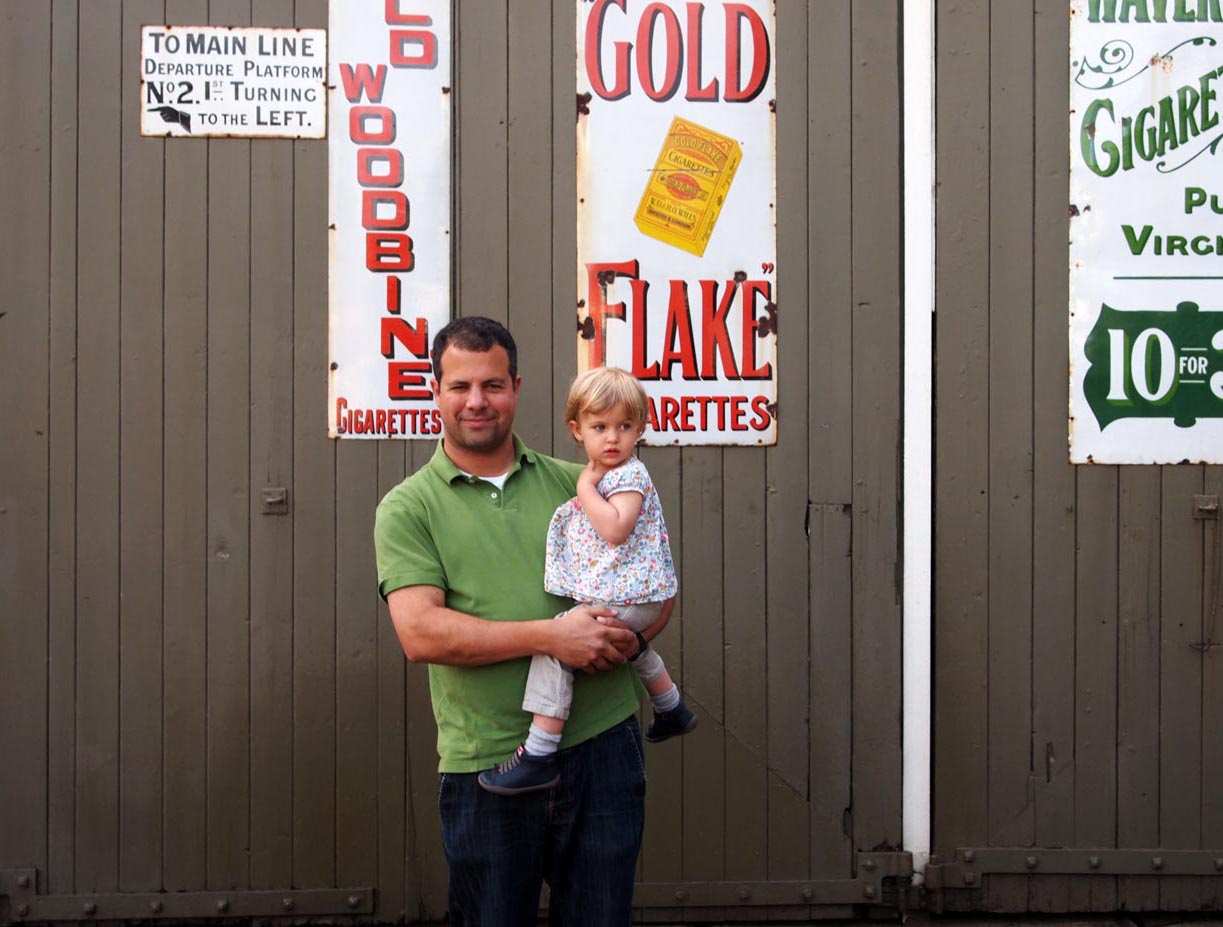In the photograph, a man dressed in a light green polo shirt and dark blue jeans holds a toddler girl in his right arm. They are standing in front of a brown wooden gate made of thin wood panels. The toddler, who is staring to the right of the image, wears a white blouse with a furrow pattern, white pants, and dark blue shoes. The wooden gate features several advertisements: on the far left, a sign reads "2 Mainline Departure Platform North 2.1" with a leftward-pointing hand symbol; next to it is a sign in white and red font for "Woodbine Cigarettes"; adjacent to that is another sign for "Gold Flake Cigarettes," accompanied by a yellow cigarette pack between the words "Gold" and "Flake." On the rightmost side is another cigarette advertisement, though the brand name is cut off.